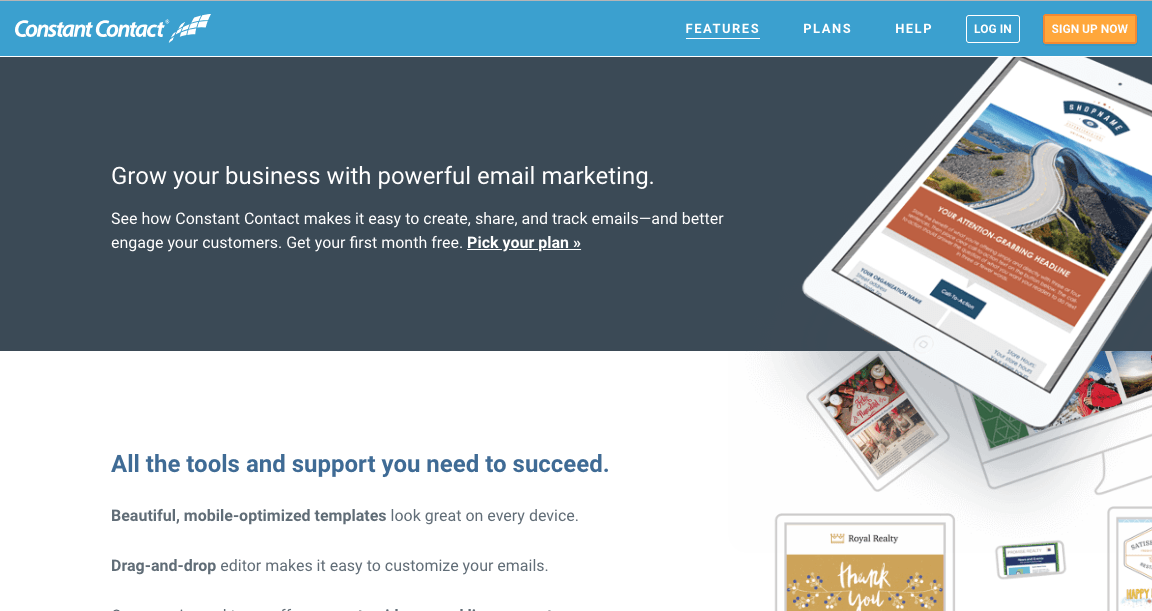This screenshot captures a detailed section of a website, featuring a complex layout with various elements:

At the very top, there is a horizontal navigation bar spanning about an inch down. The left side of the bar is light blue, adorned with the white text "Constant Contact." Positioned throughout the bar, there are groups of small squares arranged in a grid pattern: two rows at the top, four in the middle, and three at the bottom. On the far right section of the bar, there is an orange tab glowing brightly, bearing the text "Sign Up Now" in white. Adjacent to this tab is a white-outlined tab with blue text that reads "Login." Further to the left, the bar lists several options: "Help," "Plans," and "Features," with "Features" underlined.

Below this navigation bar, a section with a gray background occupies the central part of the screen. Within this gray section, approximately an inch from the left edge, white text announces, "Grow your business with powerful email marketing," succeeded by two lines of additional information. Toward the right side of this section, about two inches from the edge, a white diagonal banner extends from the top right corner downward, nearly touching the bottom. This banner appears to extend slightly out of the gray area, designed to resemble a piece of paper, possibly demonstrating a webpage design. Overlaying this banner are smaller rectangles, one to the left and another to the bottom right, partially visible.

In the white portion underneath this gray section, around three inches below the main header, additional white text reads, "All the tools and support you need," followed by two more lines of supporting text. The intricate design and careful placement of these various elements collectively provide a comprehensive overview of the website's features and offerings, emphasizing functionality and accessibility.